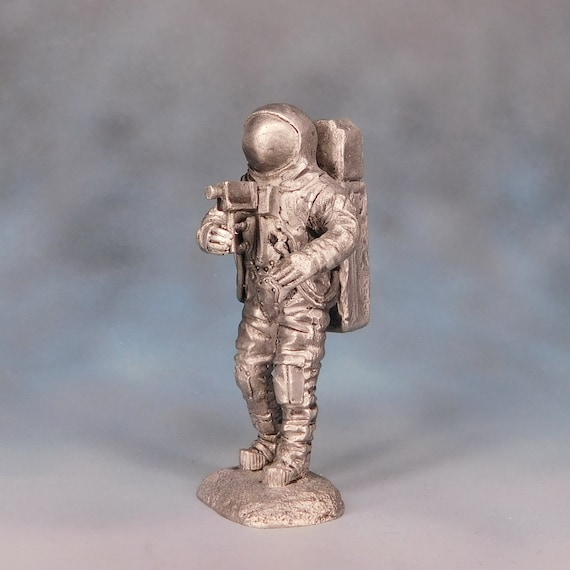The image depicts a detailed, small metal sculpture of an astronaut in a realistic spacesuit, primarily silver in color, standing on a base resembling the rocky lunar surface. The astronaut, facing left, holds a camera up to its chest, reminiscent of the iconic Hasselblad used by Neil Armstrong during the Apollo missions. The sculpture, appearing to be carved from a single piece and polished to a reflective sheen, intricately captures the suit's wrinkles and curves, conveying a lifelike quality. The astronaut's large backpack, presumably carrying air and other equipment, adds to the authenticity. The visor is smoothly curved, rendering the astronaut's face invisible. The backdrop of the image is a blurry, greyish-blue gradient that occupies most of the frame, emphasizing the statuette's intricate details.